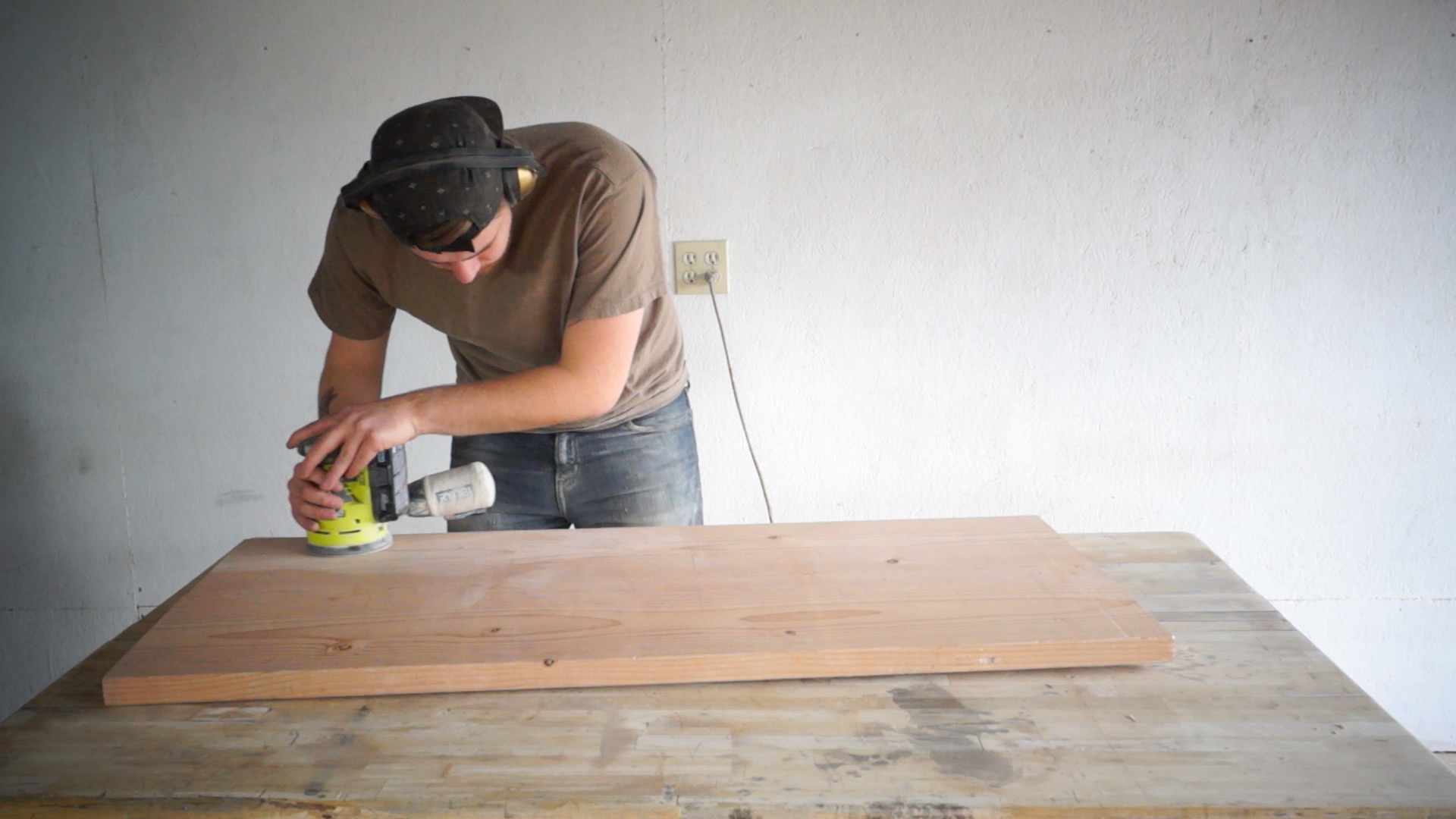In the image, a room with a gray wall serves as the backdrop. At the center of the wall is an electrical outlet with a cable plugged into it, trailing down to the floor. In the foreground, a wooden table occupies the space, and on it rests what appears to be a wooden door panel. This door panel is about half the size of the table and is made of a darker, reddish wood. On the other side of the table stands a man wearing a baseball hat turned backward and headphones over his ears. He is dressed in a brown short-sleeved shirt and blue jeans. The man is using a yellow and black sander, with his right hand positioned on the side of the sander and his left hand on top. The sander features a white cylindrical component extending from its right side.